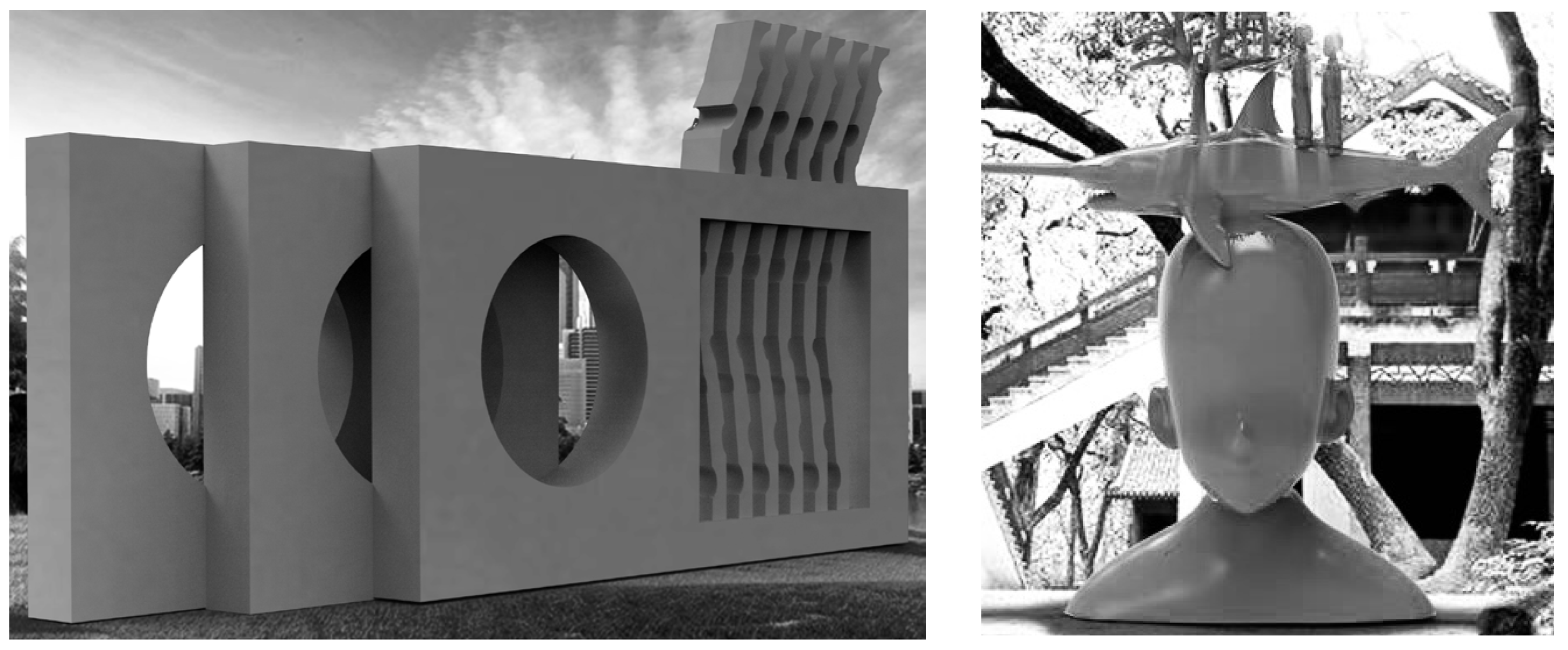This is a two-panel image, likely set in an art museum or a public park. Both panels are in black and white, predominantly in shades of gray. The left panel features three staggered rectangular structures with a textured, almost organic form protruding from the front block. Each rectangle has a circular hole on the left and a square cutout on the right, creating an abstract, architectural aesthetic set against a cement ground under a partially cloudy sky. To the right, the image depicts a statue of a child's shoulders and head, with a marlin perched on top. The marlin has a long nose, sharp teeth, and prominent fins. Behind this sculpture, a staircase and a pavilion are faintly visible, suggesting the scene is also outdoor.